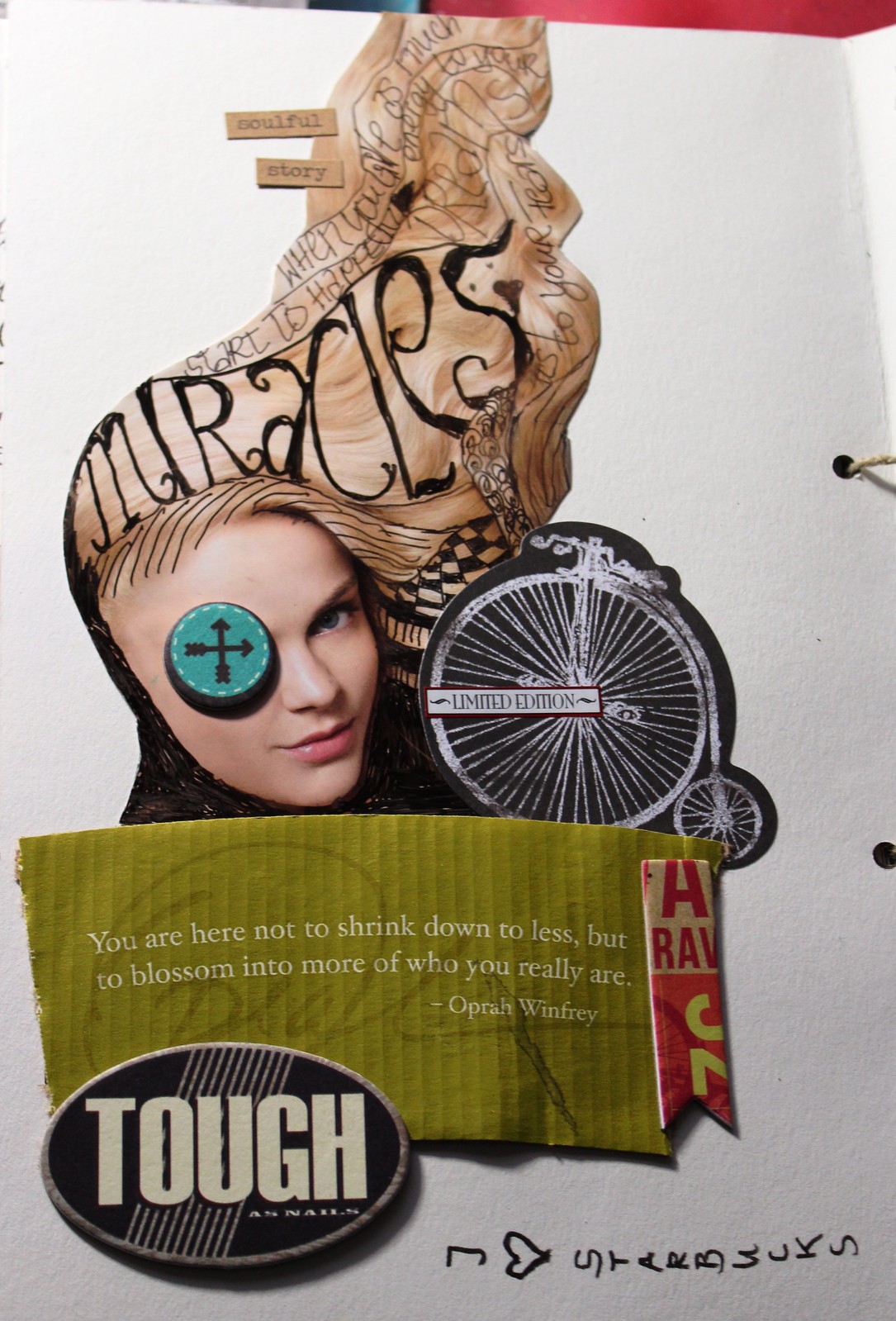This image features an intricate collage with multiple elements woven together, highlighting both abstract and textual details. At the center of the composition is a blonde-haired woman positioned towards the top-left, with hair styled upwards in waves. Notably, her right eye is replaced by a coin-like object emblazoned with two directional arrows, while her left eye and the rest of her face remain natural, albeit with a slight frown. To the right of her head is an illustration of an old-fashioned, penny-farthing bicycle labeled with the text "limited edition."

The collage also includes several distinct text elements. Below the woman's image, there is an inspirational quote by Oprah Winfrey that reads, "You are here not to shrink down to less, but to blossom into more of who you really are." This quote is attributed directly to Oprah. Additionally, there's a stamp-like emblem in the bottom-left corner with the bold statement "tough as nails," set against a black background with white stripes. Towards the lower section of the image, handwritten text proclaims, "I love Starbucks." Adjacent to the woman’s flowing hair, there's a caption that reads “soulful story,” with the hair rendered in colors that are somewhat indistinct.

Altogether, the image appears to be a creatively assembled collage with a style that merges retro and modern elements, blending motivational text with eclectic visuals for an evocative artistic effect.